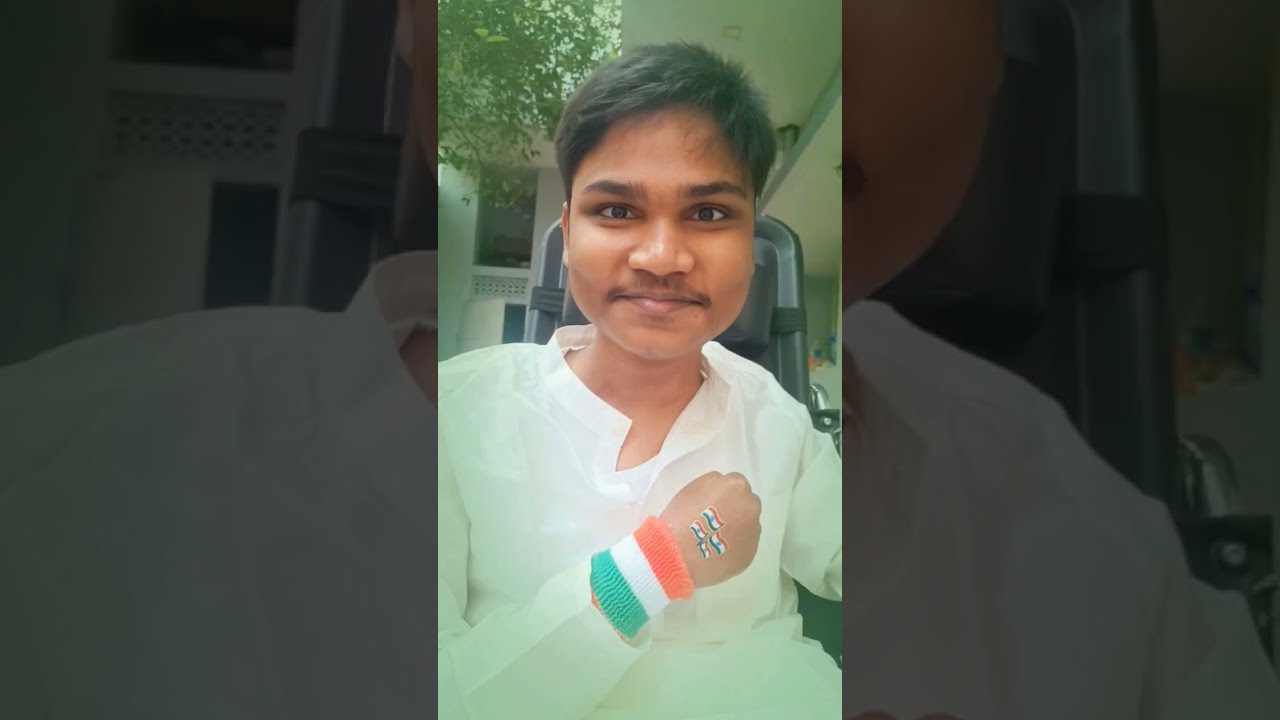The photograph appears to be a vertical selfie likely taken on a smartphone, recognizable by the characteristic black or darkened areas on either side of the central image. It features a young man, possibly in his mid-teens, with short black hair, wearing a white shirt with a U-shaped open collar. His right arm is raised with a fist clenched over his chest, displaying four temporary tattoos of the Indian flag and a wristband in the colors of the Indian flag (orange, white, and green). The setting seems to be a mix of indoors and outdoors; while the lighting and greenery over his right shoulder (our left) suggest an indoor setting, the white awning and the hint of a tree behind him give an impression of an outdoor courtyard. The young man is looking directly at the camera and appears to be smiling, with a small mustache adding to his appearance.